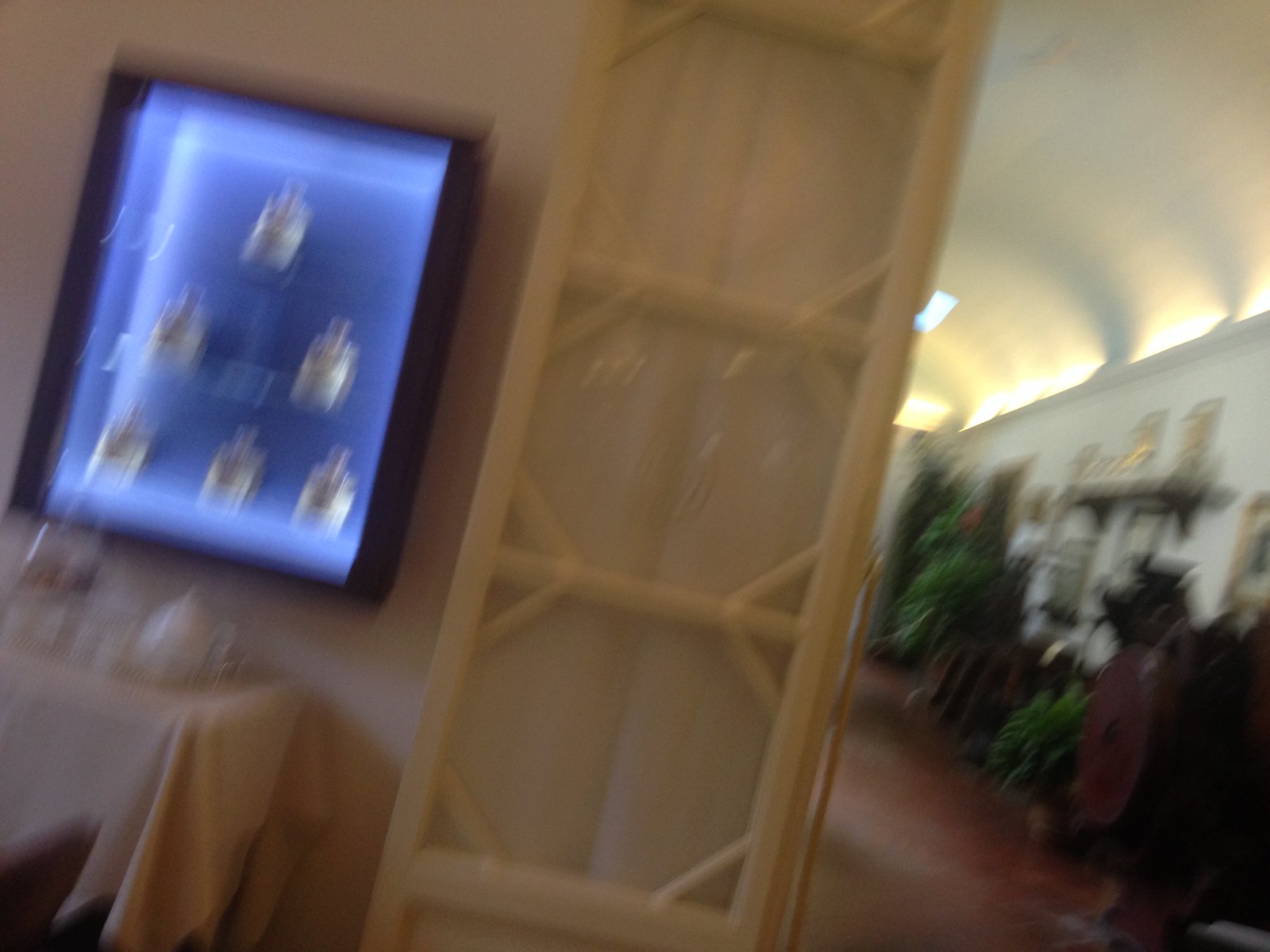The image captures a somewhat blurred and slightly tilted scene centered around a striking blue neon-lit framed display case. Inside the illuminated frame, various bottles, potentially perfume vials, are meticulously arranged, drawing the viewer's attention. Beneath this ornate display, a small table draped with a tablecloth showcases a delicate tea service set, adding a touch of elegance to the area. To the left of the setup, a shelving unit crafted from bamboo or light-colored wood acts as a subtle divider. To the right, the space opens up into a vast area filled with abundant greenery and foliage, leading up to a gracefully curved roof, merging natural elements with refined decor.